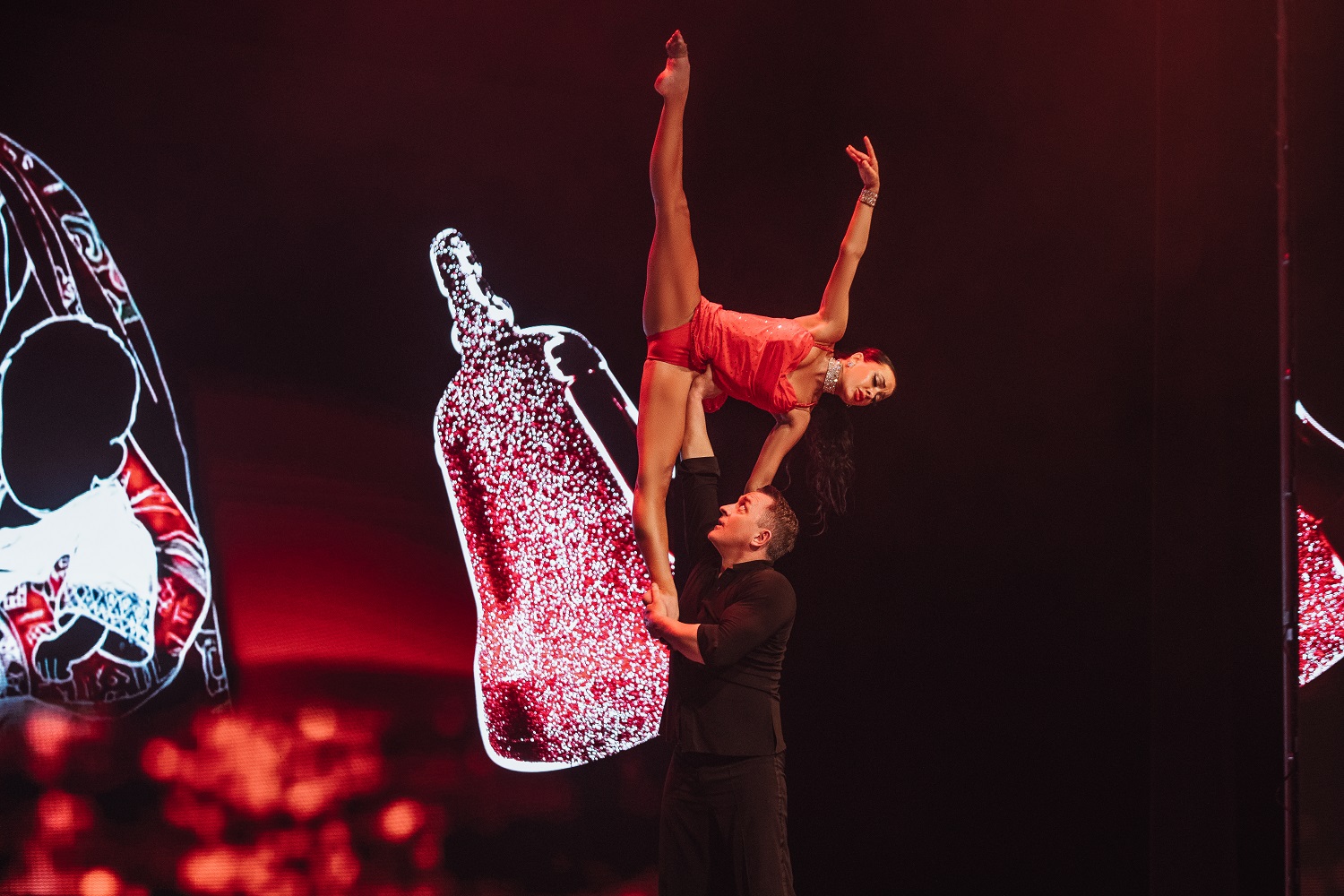In the center of the stage, a man dressed in a black button-down shirt and black pants stands in profile, lifting a woman high off the ground. The woman, clad in a vibrant red leotard resembling a bathing suit and adorned with a sparkling diamond necklace, has short, dark hair that flows behind her due to the dynamic movement. Supported by the man's right arm at her waist and his left hand holding her left foot, she strikes an elegant pose with her right leg fully extended in a straddle and her arms curved gracefully above his head. The stage is set against a moody, dramatic backdrop, with the left side featuring a reddish hue that transitions into a dark, starry or bokeh-like pattern, punctuated by bright, speckled designs that resemble stylized Christmas bells. A stark black curtain frames the right side of the scene, enhancing the contrast and theatrical ambiance of their acrobatic dance routine.